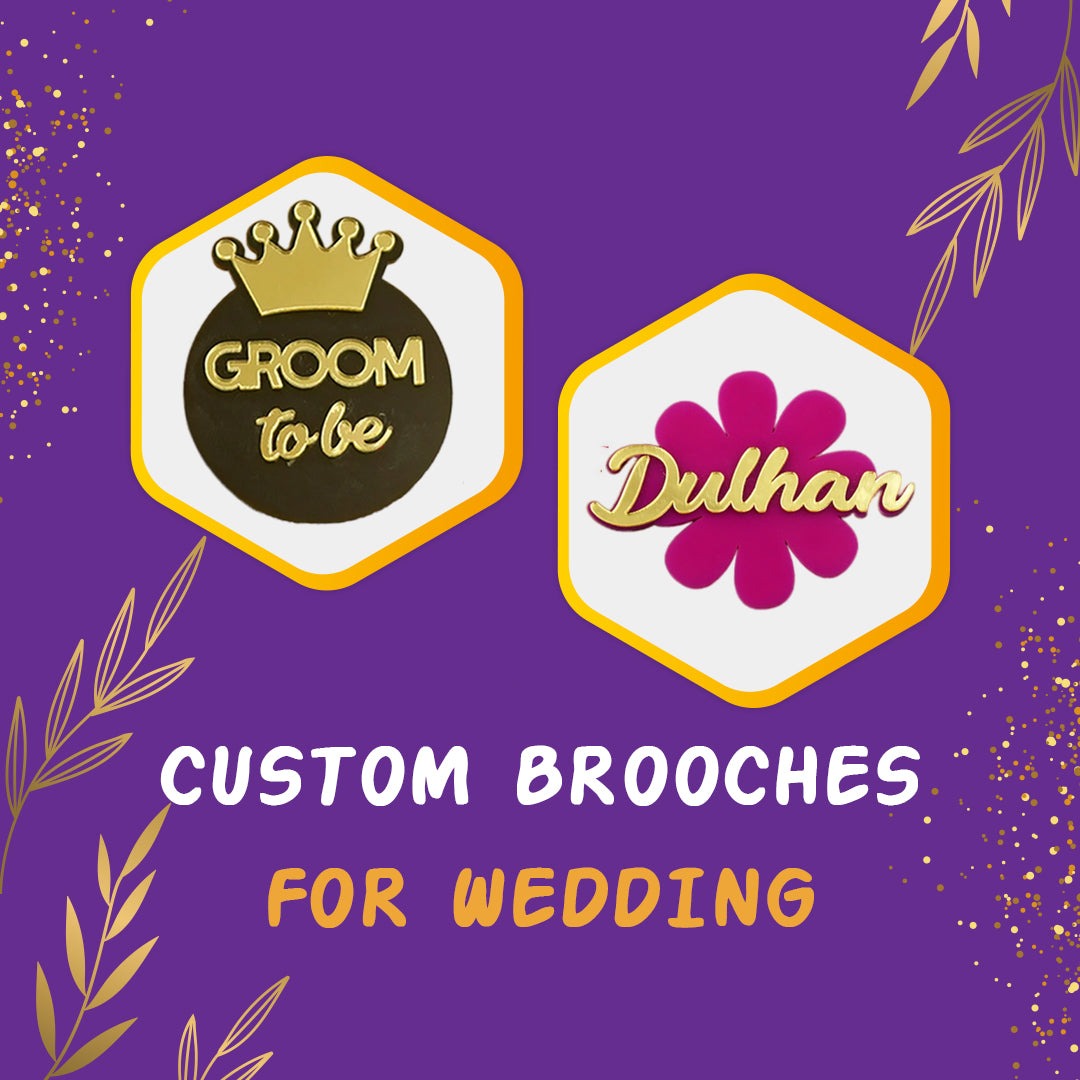This image is a square-shaped advertisement with a flat purple background featuring gold foil embellishments that resemble a faux glitter effect. The gold embellishments are situated in the upper left and lower right corners. Additionally, the upper right and lower left corners showcase stylized gold branches with leaves. Central to the image are two prominent eight-sided shapes, each set on a point. One shape contains a black circle with gold writing that reads "Groom to Be" and is topped with a crown. The other contains a pink flower with gold writing that reads "Dulhan." Below these shapes, it states "Custom Brooches for Weddings" in white print. This image serves to showcase the types of brooches available from this company.